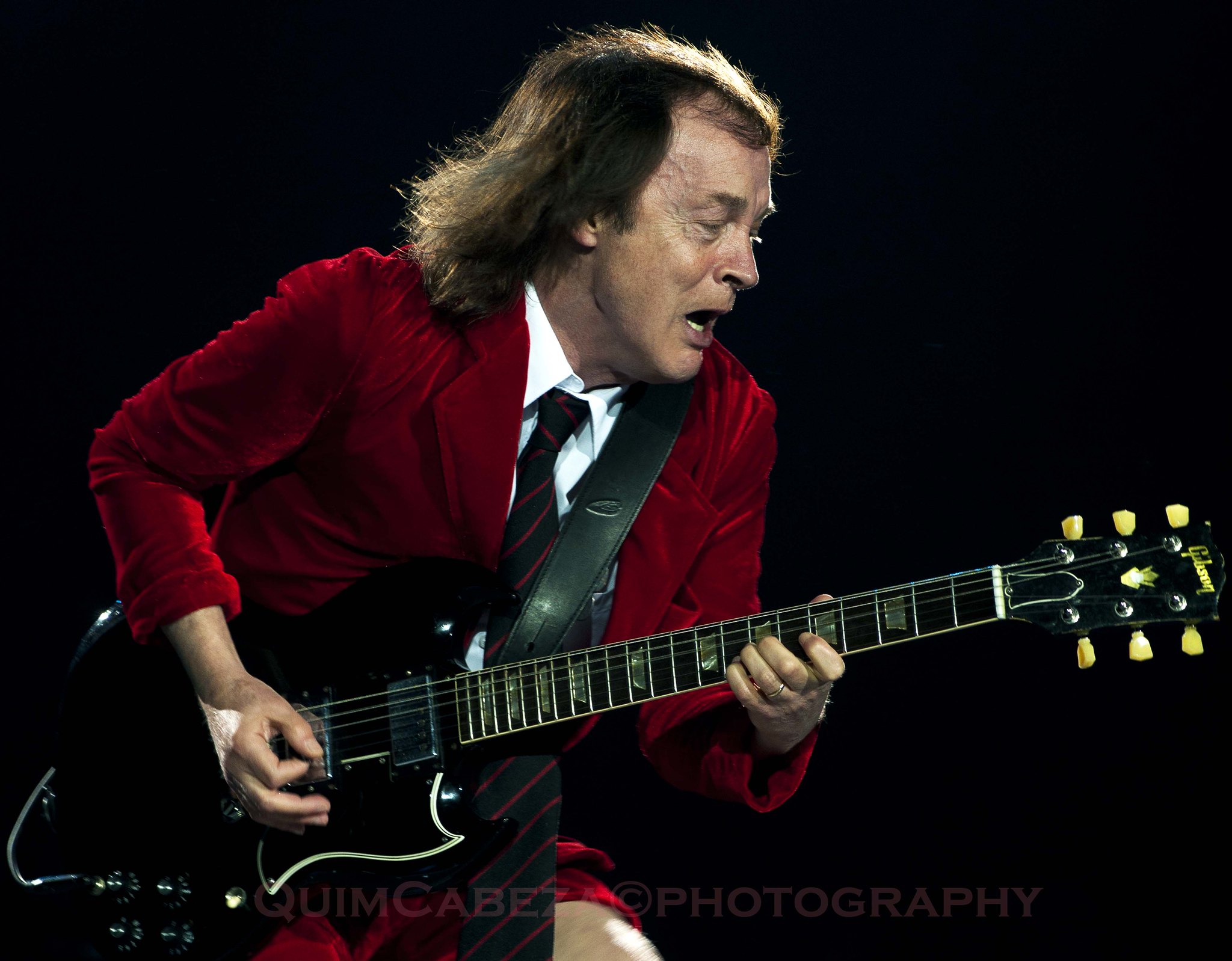In this image, we see an older, middle-aged man performing, slightly left of center, in a dimly lit or outdoor setting characterized by an all-black background. He is wearing a red velvety suit coat over a white shirt, paired with a dark tie featuring red stripes. His longish brown hair drapes down to his shoulders, particularly noticeable on the right side, as he faces slightly to the right with his mouth open, possibly singing. The man is playing a black guitar, supported by a black strap over his left shoulder, with his right hand strumming and his left hand on the chords. The guitar and parts of his outfit introduce a range of colors including black, brown, tan, red, silver, gold, and maroon. A hint of red beneath the guitar suggests either his outfit or pants, partially visible alongside his tie. The composition is centered around him, with the black background providing a stark contrast to his vibrant attire. At the bottom of the image, the watermark "Quim Cabot Photography" subtly appears. The setting seems to depict a concert scene.